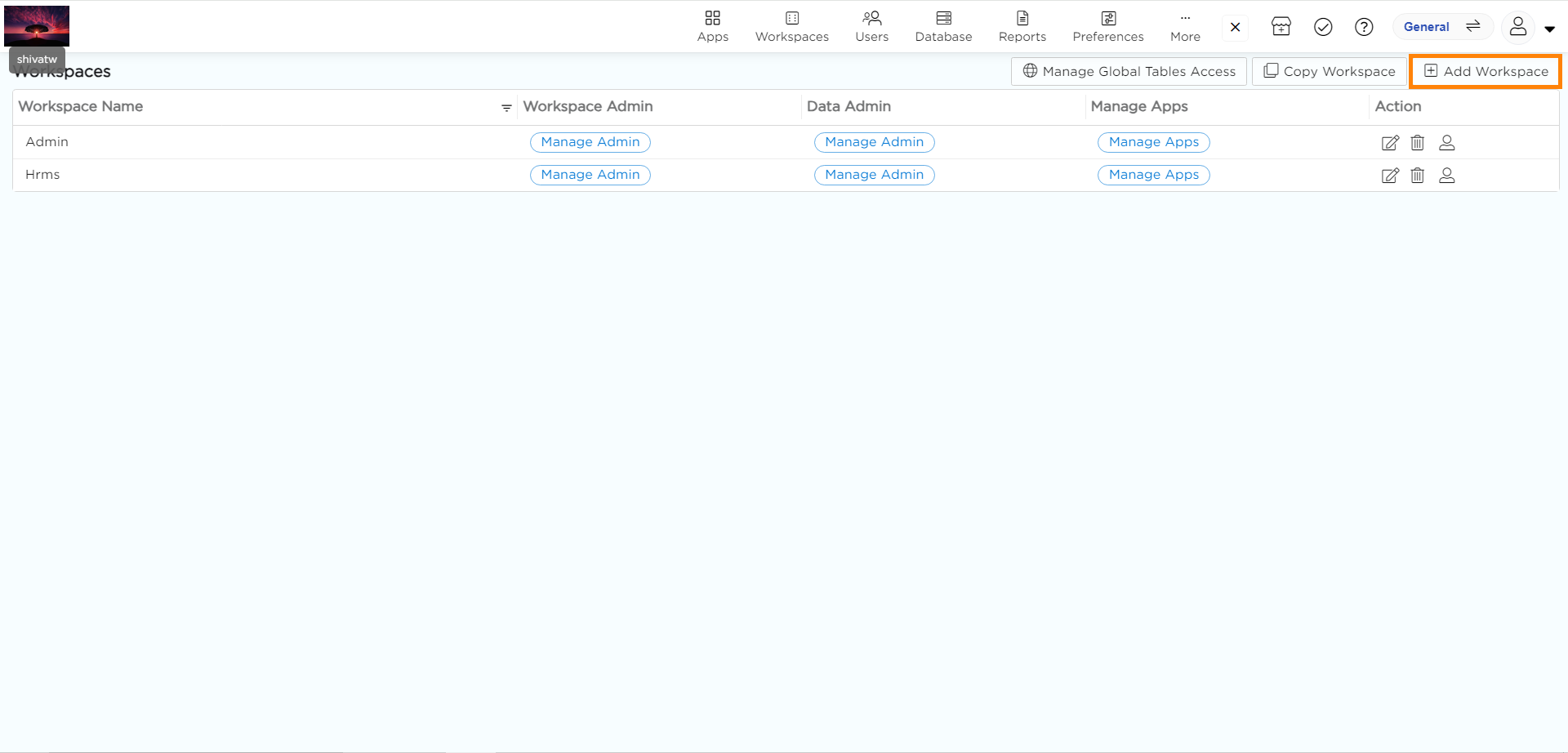This is a detailed screenshot of a settings page on a website. At the top, there is a white header featuring a photograph of a sky and ocean scene with a pink and orange hue located in the top left corner. Below this image, a small hovering panel displays the text "Shiva TW." On the right side of the white header, there is a row of labeled icons, organized from left to right: Apps, Workspaces, Users, Database, Reports, Preferences, and More. To the immediate right, there is an 'X' icon followed by additional icons, including a shop kiosk, a checkmark, a question mark, a pill-shaped button with "General" written in blue text, and a generic profile picture icon.

Below the white header, the page background transitions to a pale blue, creating a spacious area with significant negative space at the bottom. At the top of this section, there are two lines of information set against a white background. The page is titled "Workspaces," with three buttons to the right of this title: "Manage Global Tables Access," "Copy Workspace," and an orange-highlighted "Add Workspace" button.

The section below these buttons features a table with headers labeled as "Workspace Name," "Workspace Admin," "Data Admin," "Manage Apps," and "Action." Under these headers is a row labeled "Admin," accompanied by blue buttons to the right that say "Manage Admin," "Manage Admin," and "Manage Apps." Another row follows labeled "HRMS," which includes similar blue buttons for management options.